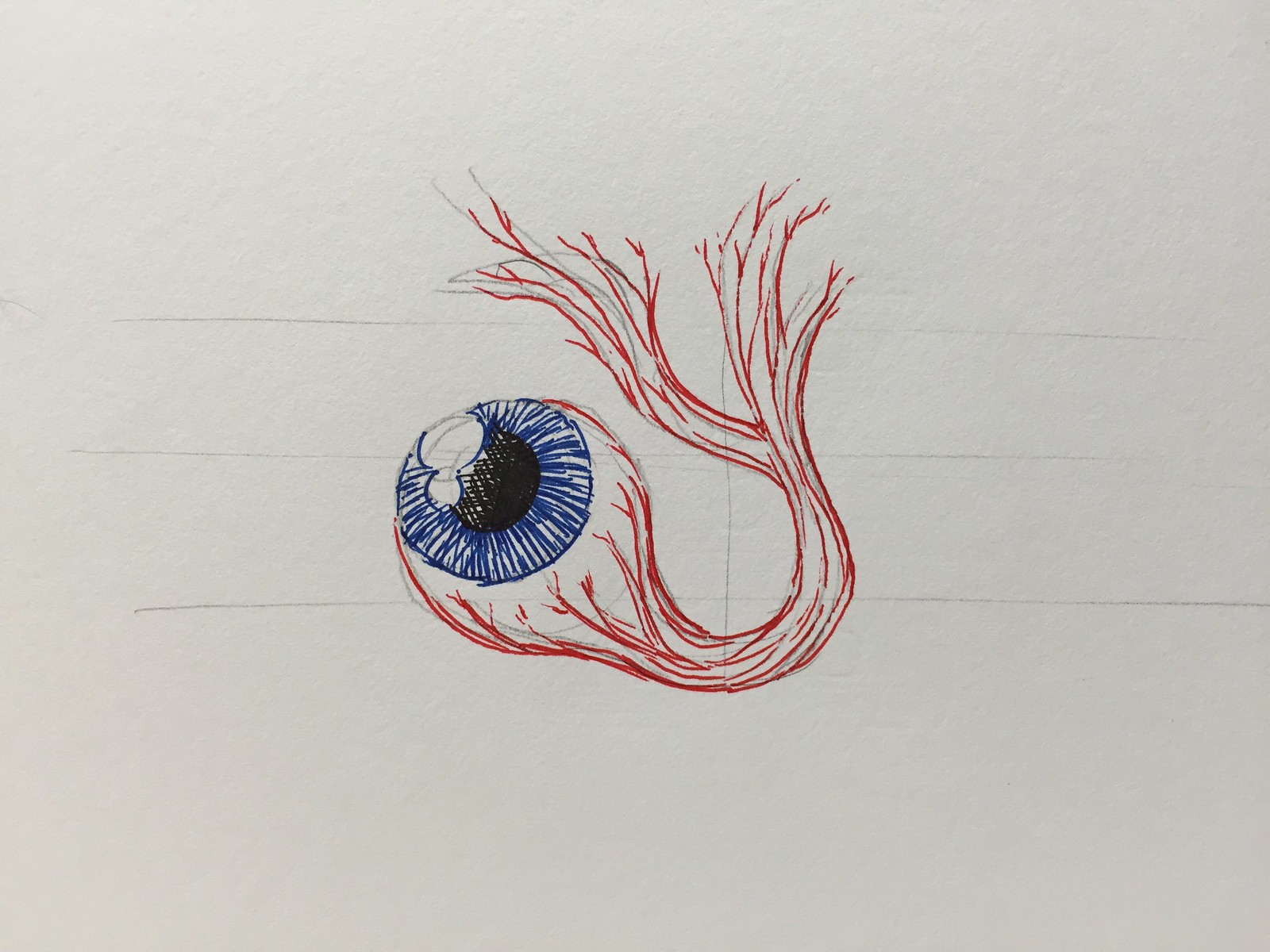This image is a detailed and striking photograph of a meticulously crafted drawing, rendered on what appears to be textured white sketchbook paper or cardstock. The central subject is a highly graphic depiction of a human eyeball, featuring a blue iris and a large black pupil accented with two reflective eye spots. The drawing medium includes both ink, likely from a gel pen or ballpoint pen, and pencil, which is used for underlying guidelines visible in the background. These guidelines help in precisely placing the artistic elements. The eyeball itself is completely round, not housed within any face, and appears to be plucked out, giving it a surreal quality. Extending from the back of the eyeball are vividly drawn blood vessels or tendons, depicted in red ink. These veins are notably detailed, starting from the white of the eye, then twisting and splitting into two sections, creating a dynamic, almost three-dimensional effect against the textured white background.